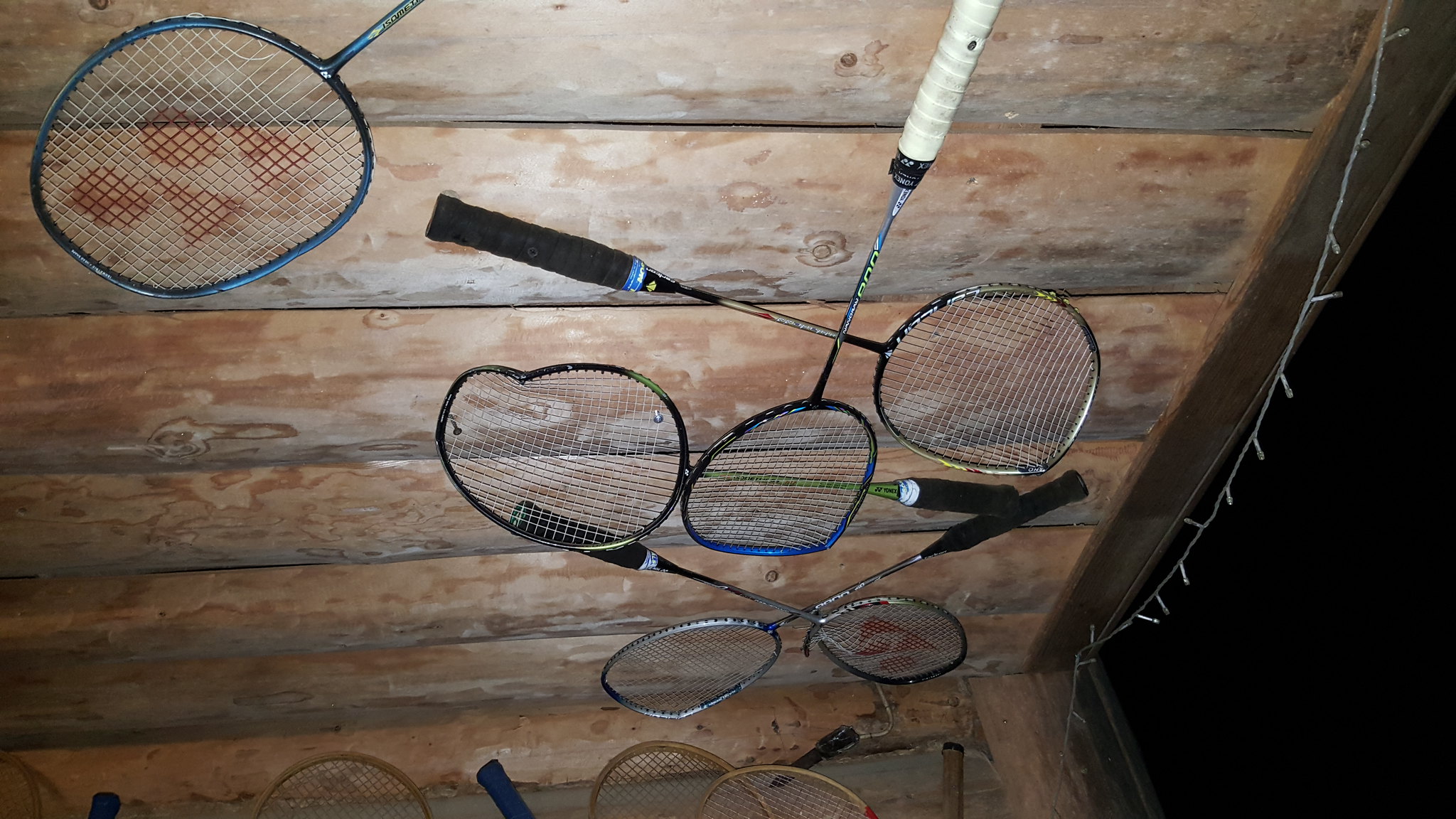The photograph captures a dimly lit scene, likely taken at night with a flash, showcasing an old, worn wooden wall. The wall's surface, which might initially appear as a ceiling due to the camera angle, is constructed of untreated or lightly varnished wood beams. Adorning the right side of this wall is a string of unlit, white Christmas lights. Scattered haphazardly and nailed to the wooden surface are numerous badminton rackets in various states of disrepair. There are at least six visible on the main wall, with additional ones partially seen on another overlapping wall section. These rackets showcase significant wear: many are misshapen, with dented frames and damaged strings. Some rackets feature black handles while others have white, and notably, one has red paint markings. The overall arrangement and condition of the rackets suggest they have been neglected or poorly treated, transforming them into mere debris against the rustic wooden backdrop.